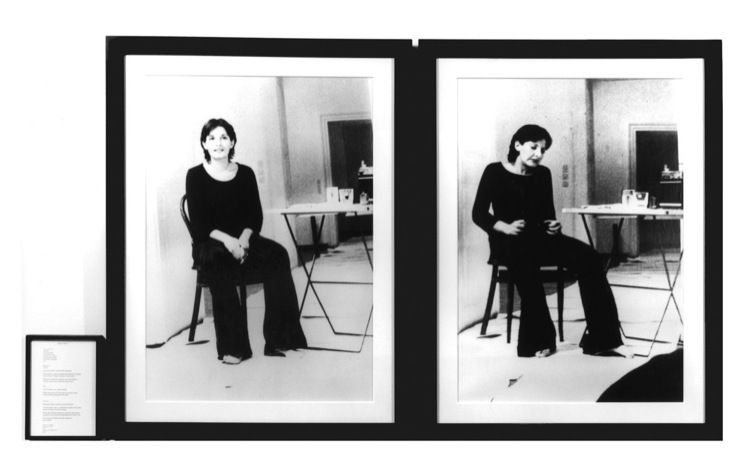The image displays two side-by-side, black-and-white photographs set against a white background, each encased in a thick dark frame with a white mat. Both photos capture the same woman seated in a chair within a room characterized by light flooring and white walls. She has short black hair reaching her neck, and she wears a long-sleeved black top paired with loose, belled black pants, remaining barefoot in both images.

In the left photograph, the woman sits with her hands in her lap, gazing directly at the camera. In the right photograph, she looks slightly downwards toward the bottom right. Positioned beside her is a folding table holding various indistinguishable items, possibly including glasses and a radio. Behind the table, a doorway can be seen in both images.

Both photos are uniformly spaced in the center of the overall composition, with what appears to be a small white piece of paper carrying text, likely detailing the photographs or exhibit, in the bottom-left corner of the image. The overall setting suggests the photographs are part of an art exhibit, hanging neatly on a wall.